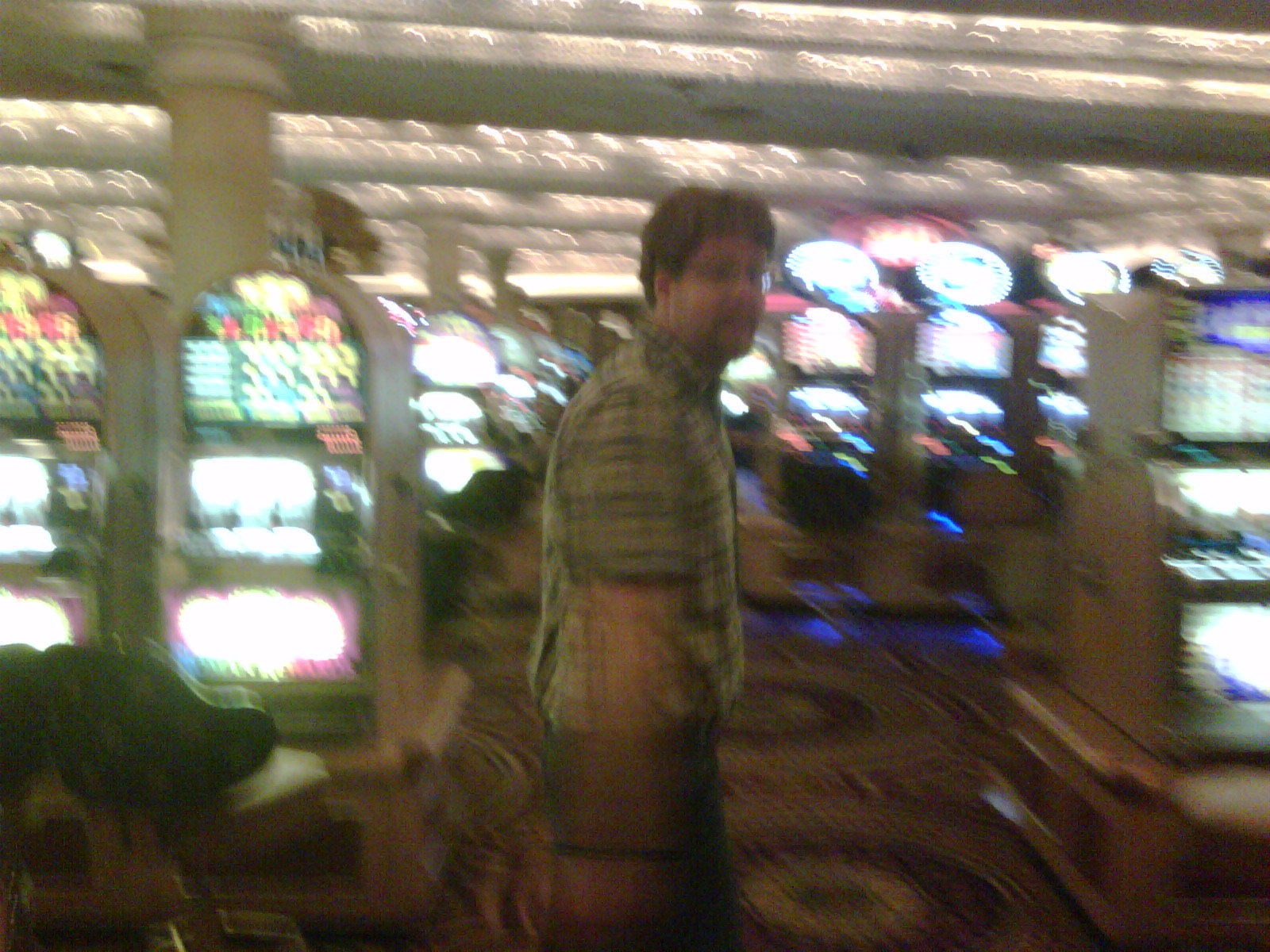In this blurred photograph taken inside a lively casino, a man with short brown hair, glasses, and a goatee is the focal point. He is captured mid-step, conveying a sense of motion, which adds to the overall blurriness of the image. The man is positioned in the center of the frame, standing amidst an array of slot machines that stretch into the background, their bright lights contrasting with the subdued palette of the floor and walls. He is wearing a yellow and darker plaid short-sleeved shirt, tucked into grey pants with a belt. The casino's ceiling is adorned with bright lights, and there are off-white columns positioned to the left of the man. The carpet underfoot is brown with circular patterns, complementing the greyish border blocks around the standing man. Despite the overall brown tone of the photograph, the lights from both the ceiling and slot machines illuminate the scene, highlighting the bustling, vibrant ambiance of the casino. The man's body slightly faces to the right, but his head turns towards the camera, giving the impression he is aware of being photographed.